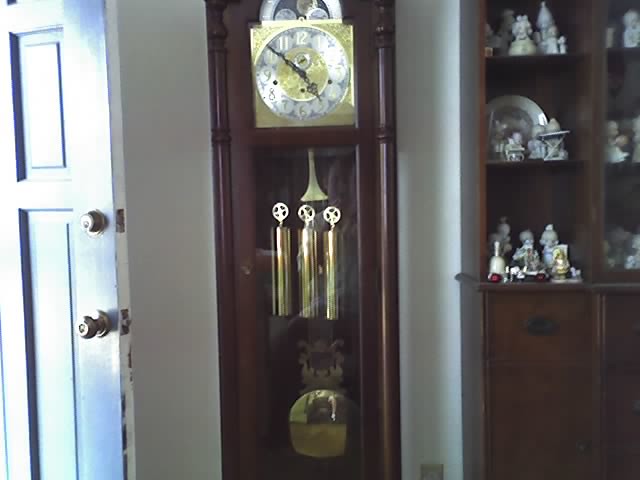A stately grandfather clock stands elegantly next to an open blue metal doorway, its intricate design captivating in rich, dark cherry-colored wood. The face of the clock, encased in a gold-colored square, features a silver background adorned with black numbers circled elegantly, with a unique distinction of white numbers towards the top. At its center, a golden interior houses the hour and minute hands, adding a luxurious touch to its appearance. Below the face, shiny brass weights and a pendulum gleam, marking the time at 4:50. Above the clock face, a silver arc with three discs adds a sophisticated flair. To the right of the clock, a china cabinet displays an assortment of fancy knickknacks, complementing the sophisticated ambiance of the room.